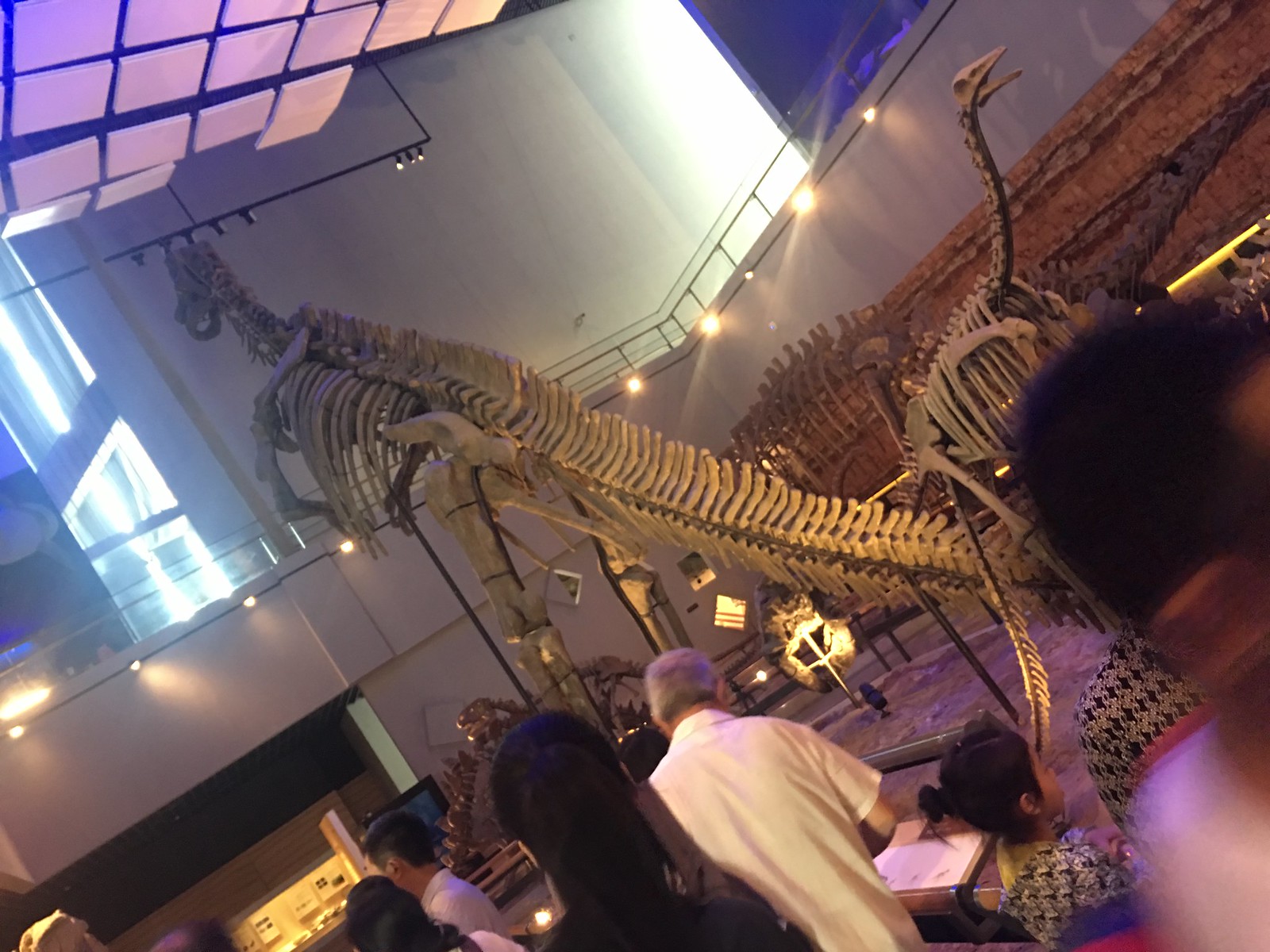This is a photograph taken inside a museum, showcasing a dinosaur skeleton exhibit. The image appears to be taken at an angle, giving it a diagonal and almost topsy-turvy perspective. Dominating the center of the photograph is a large, white dinosaur skeleton, possibly with long arms and a shorter head, its bones artistically lit to contrast with the ambient lighting of the room. The backdrop features a mural depicting the land these creatures once roamed. Below the skeleton, visitors, predominantly of Asian descent, are engaged in reading informational plaques at the base of the exhibits. Some of the visitors appear blurred due to movement, adding a dynamic quality to the scene. The room boasts a high ceiling with a skylight, allowing natural daylight to filter in, complemented by artificial lighting from a surrounding balcony, which casts a soft purplish hue over the scene. In the lower right corner, a man can be seen, possibly overseeing the exhibit or providing information to the guests.